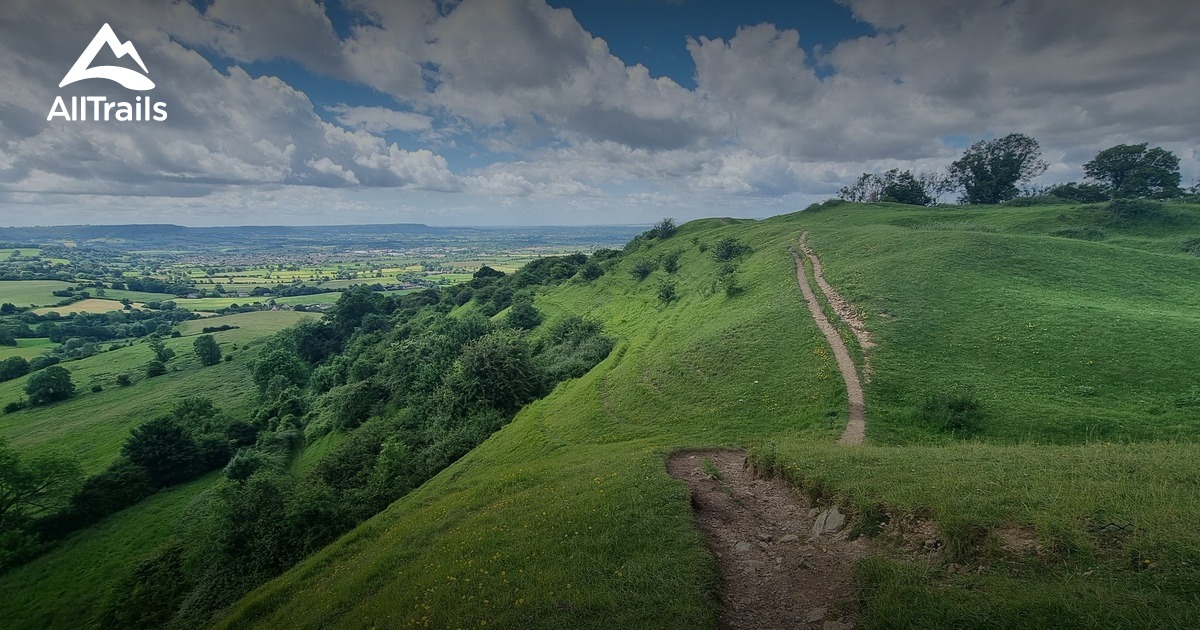The image captures a picturesque landscape showcasing a well-worn, narrow dirt trail situated on the right half of the frame, extending into the distance. Surrounding the trail, gently rolling green hills are adorned with short grass, wildflowers, and clovers, gradually becoming more wooded ahead and to the left. The left side of the image features a slope descending into a wide, flat region dotted with various large fields and sporadic trees. The bright blue sky is sprinkled with many large, fluffy white clouds. In the top left corner, a stylized logo depicting a mountain is present, accompanied by the text "All Trails" beneath it. The overall scene exudes a clean, verdant aesthetic with vibrant green foliage and scattered patches of dirt, capturing a serene and inviting natural environment.